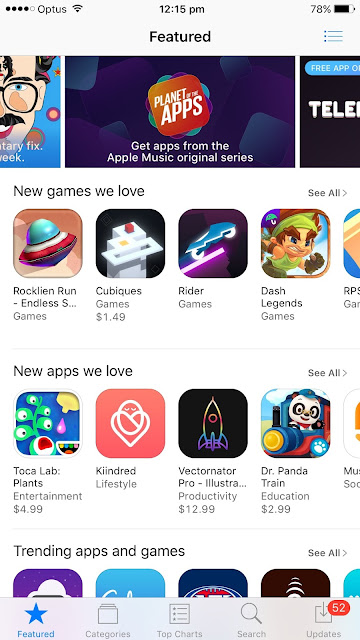In this image, we see a smartphone screen displaying an app store interface. 

**Top Bar:** 
- The top-left corner features a status bar with four black dots, one clear dot, the "Optus" network indicator, and a Wi-Fi icon.
- The top-right corner displays a battery percentage of 78%.

**Time and Headings:** 
- The center of the screen shows the time as 12:15 p.m.
- Below the time, the main heading reads "Featured."

**Sections and Categories:** 
- There are three main categories listed: "New Games We Love," "New Apps We Love," and "Trending Apps and Games."

**App Listings:**
- Under "New Games We Love," four apps are visible with part of another app displayed:
  1. *Rocklin Run Dash Endless S* (categorized under Games)
  2. *Cubicues* priced at $1.49
  3. *Rider*
  4. *Dash Legends*

- In the middle section titled "New Apps We Love," the displayed apps are:
  1. *Tokolab Plants* priced at $4.99
  2. *Kindred*
  3. *Vector Mater Pro* priced at $12.99
  4. *Dr. Panda Train* priced at $2.99

- Below this section, under "Trending Apps and Games," only the top portions of the app thumbnails are visible:
  1. The first thumbnail on the left, which is purple and white
  2. The middle thumbnail, which is blue
  3. The next thumbnail to the right, which is dark blue
  4. The last visible thumbnail, which is dark brown.

**Footer:**
- The bottom of the screen contains five navigation icons:
  1. "Featured" marked with a blue star
  2. "Categories"
  3. "Top Charts"
  4. "Search"
  5. "Updates" with a red notification badge indicating 52 updates.

This detailed layered structure provides a comprehensive view of the application store's main page.